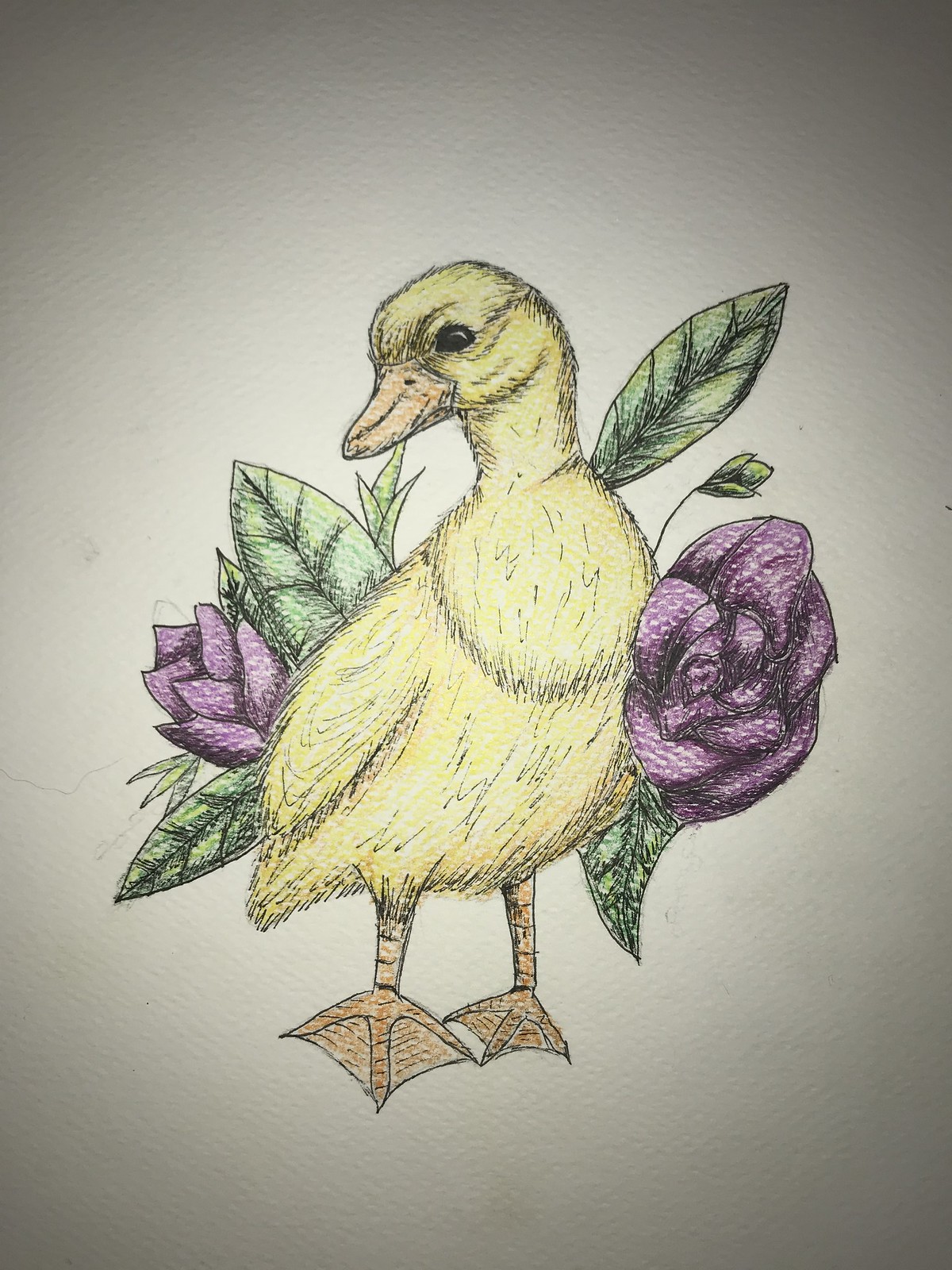This photograph captures a beautifully detailed drawing on a slightly textured sheet of white cardstock paper. The focal point of the artwork is an intricately rendered duckling. The duckling's large black eye, highlighted to convey a sense of liveliness, contrasts strikingly with its orange bill. Its downy yellow plumage is meticulously shaded, giving it a soft, fluffy appearance. The duckling stands on its orange, webbed feet, which are also depicted with attention to detail. Surrounding the duckling are elements of nature; to the right, a fully bloomed rose, and to the left, a budding rose, both accompanied by several lush green leaves and blades of grass. These elements add depth and context to the scene, suggesting the duckling is in a natural setting. The entire image appears to be skillfully colored using colored pencils, adding richness and texture to the drawing.